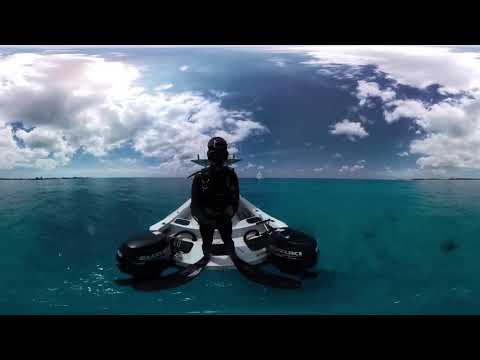The image depicts an outdoor scene of a person, presumably a diver, on a small white watercraft equipped with two large black outboard motors. The individual is dressed in an all-black diving suit with matching large flippers and is situated towards the back of the boat. The photo, taken with a somewhat distorted, possibly fisheye lens, shows the diver from an unclear angle, making it difficult to discern facial details or whether they are facing the camera. The scene is set on a dark blue ocean, under a partly cloudy sky with the sun nearly overhead. In the distant background, landmasses are faintly visible. The image is not sharply focused, and there's a noticeable black spot on the camera lens. The sky features a mix of blue shades and various cloud formations, contributing to the overall vibrant yet serene maritime atmosphere.